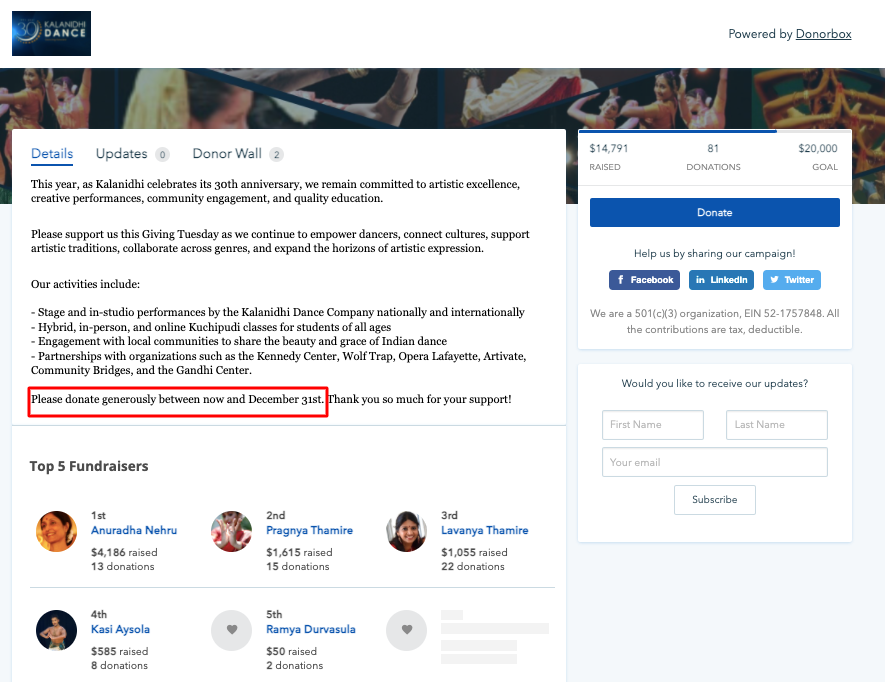The website in the image is dedicated to a dance organization, and although the site's name is somewhat unclear, it is powered by DonorBox. The background features a vibrant scene where numerous people are swirling and dancing energetically, capturing the spirit of the event.

In the foreground, there are two prominent pop-up screens. The larger pop-up on the left is focused on providing various tabs labeled 'Details,' 'Updates,' and 'DonorWall,' with the 'Details' tab currently selected. This detailed section highlights the 30th anniversary celebration of Kalindi, emphasizing their commitment to artistic excellence, creative performances, community engagement, and quality education. The text calls for support on Giving Tuesday to continue empowering dancers, fostering cultural connections, preserving artistic traditions, collaborating across genres, and pushing the boundaries of artistic expression.

Specific activities of Kalindi include stage and in-studio performances by the Kalindi Dance Company, both nationally and internationally, as well as hybrid in-person and online Kuchipudi classes for students of all ages. There is a notable emphasis on community engagement to display the elegance of Indian dance and partnerships with esteemed organizations like the Kennedy Center, Wolf Trap, Opera Lafayette, Artivate, Community Bridges, and the Gandhi Center.

The image also highlights a fundraising appeal, showcasing the top five fundraisers and their contributions. Users are encouraged to donate generously, either supporting the overall cause or contributing in the name of specific fundraisers, facilitated through online donations.